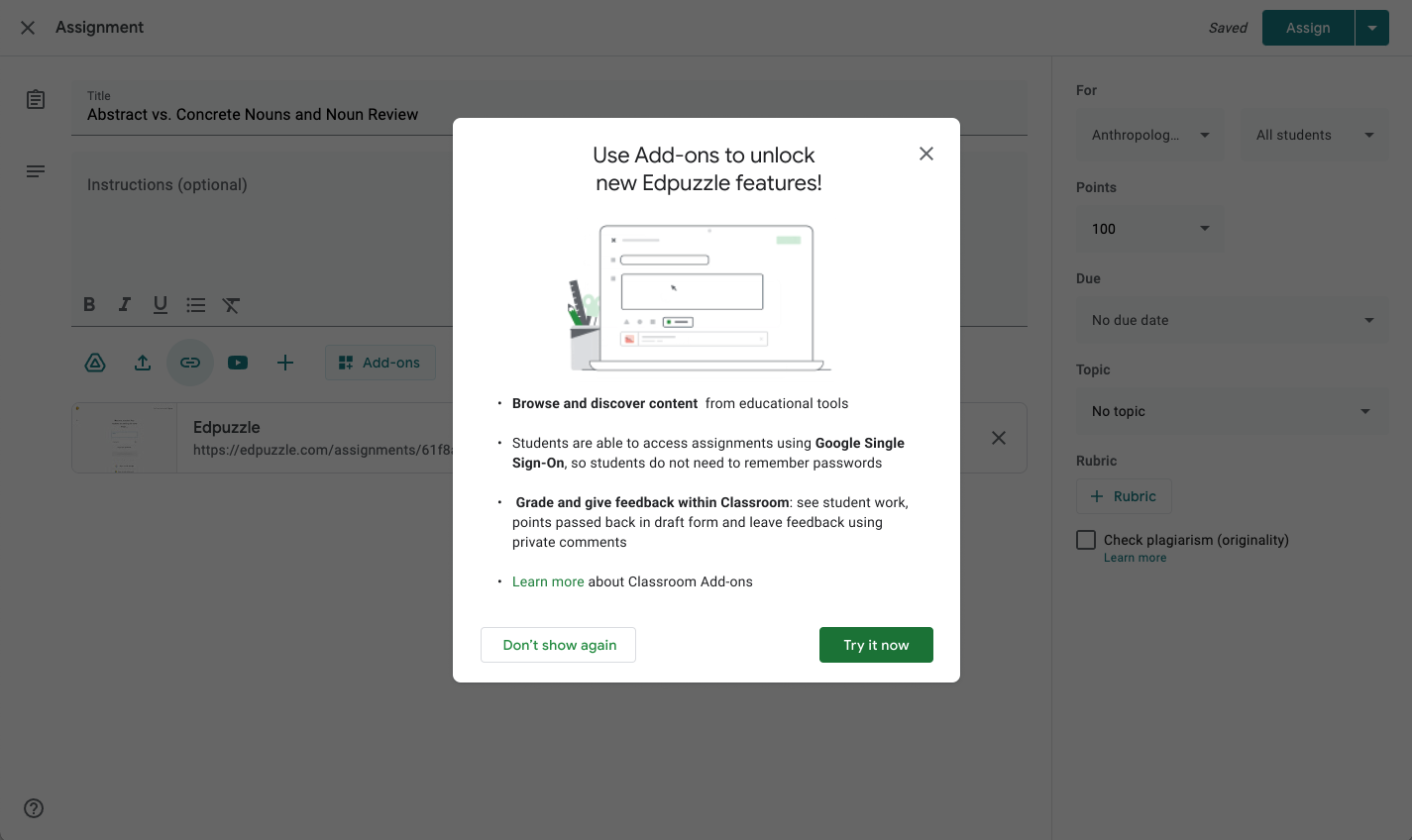A screenshot shows a pop-up window, prominently displayed against a grayish background. The pop-up is a white rectangle with a black header text stating, "Use add-ons to unlock new Edpuzzle features!" followed by an exclamation point. Below this heading, there is a hand-drawn illustration of an open laptop, with a cup behind it containing a pencil, a pair of scissors, and a ruler.

The main body of the pop-up contains four bullet points with the following features:

1. "Browse and discover content from educational tools."
2. "Students are able to access assignments using Google simple sign-on so students do not need to remember passwords."
3. "Grade and give feedback with Classroom. See student work points passed back in draft form and leave feedback using private comments."
4. "Learn more about Classroom add-ons," with the "Learn more" text highlighted in green, indicating it is clickable.

At the bottom of the pop-up, there are two action options: a white box with green text that says "Don't show again" on the left, and a green "Try it now" button on the lower right.